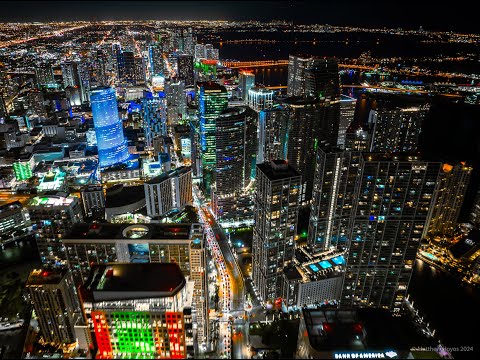This photograph captures a vibrant nighttime aerial view of a bustling downtown area, alive with colorful, illuminated skyscrapers. The cityscape is dominated by buildings lit up in striking hues, with some skyscrapers bathed entirely in blue light, while others are adorned with green and red lights along their sides. The landscape is dotted with busy roads teeming with cars and their headlights, reflecting the city's relentless energy. To the top right of the image, the reflection of water can be discerned, possibly indicating a nearby river or bay. The distant city lights shimmer faintly on the horizon, contrasting sharply against the night’s darkness. Among the brightly lit buildings, the recognizable "Bank of America" text stands out at the bottom right of the image, although some accompanying writing remains indecipherable. The photograph also features distinct arching lights indicative of bridges, adding to the urban mosaic. The overall scene encapsulates the essence of a city that is vibrant, dynamic, and very much alive.